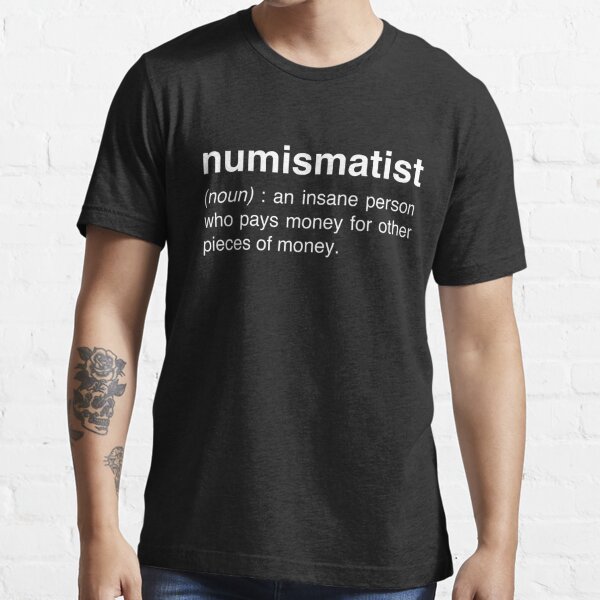This is a photo of a light-skinned man wearing a black t-shirt with white lettering. The shirt prominently displays the word "numismatist" along with its definition: "noun: an insane person who pays money for other pieces of money." The man is positioned in front of a white, painted brick wall, with the bricks being clearly rectangular. The shot captures him from just below the neck to the upper portion of his thighs, including a bit of his blue jeans. His arms, which hang at his sides, feature visible tattoos; notably, a skull and flower in dark green ink on his right forearm. The photo's composition focuses on the t-shirt's text, with the man's head being mostly out of the frame, suggesting that the primary subject is the shirt's design and message.